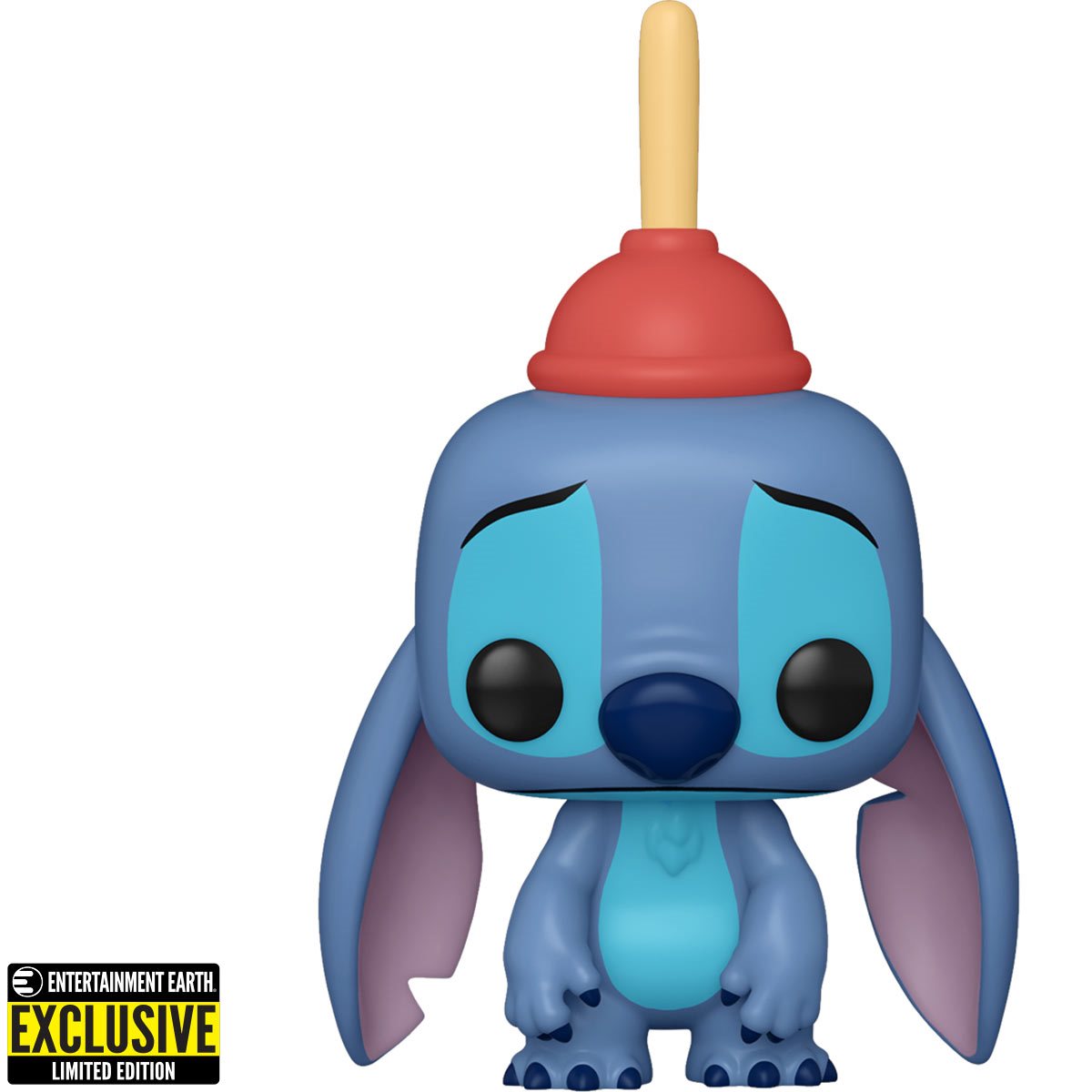The image depicts a toy modeled after Stitch from "Lilo and Stitch." The toy features Stitch with a sad expression, large black eyes with teal eyelids, and drooping, long ears that are blue with pink innards. It has a dark blue nose and a teal midsection. Notably, a light brown plunger with a yellow handle is suctioned to the top of its head, adding to its forlorn appearance. The figure's body is disproportionally smaller than its head, with short legs and small toes and fingers. The entire image has a computer-generated look. Positioned to the left, there's a black and yellow banner with the label "Entertainment Earth Exclusive Limited Edition," denoting it as a special collectible item.